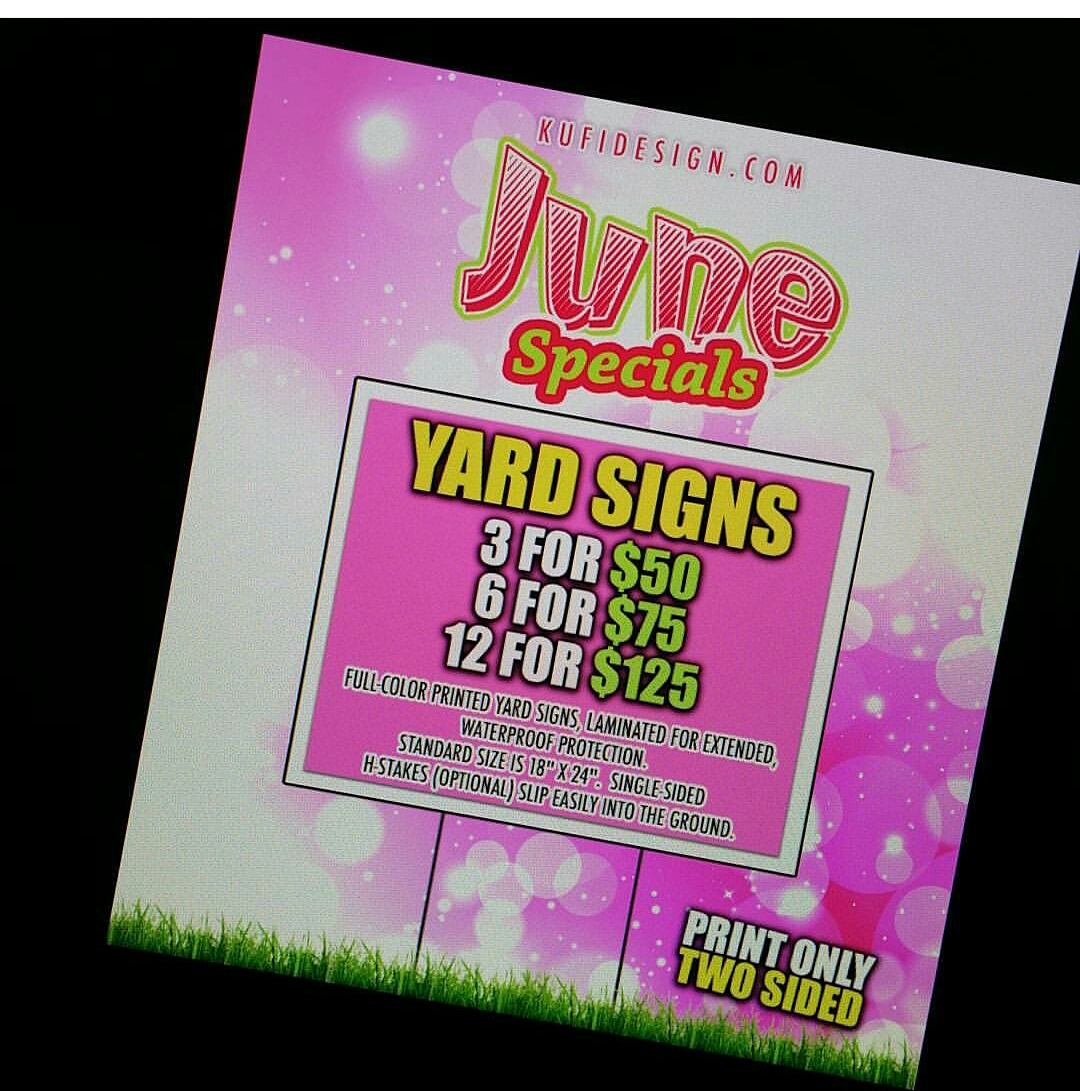The image depicts a vividly colored advertisement set against an all-black background. Central to the composition is a square-format poster dominated by bright pink and white abstract bubbles. Boldly displayed at the top in dynamic pink lettering is "KooFiDesign.com," followed by "June Specials" written in eye-catching hand-drawn pink with a green drop shadow and green text with a pink drop shadow, respectively. The main promotional content is laid out within a pink horizontal rectangle at the center, featuring the words "Yard Signs" in bold yellow letters. Below, pricing details are listed: "3 for $50, 6 for $75, 12 for $125," alongside specifics about the product – full-color printed, laminated for extended waterproof protection, and available only in two-sided print. A stylized illustration at the bottom mimics an actual yard sign with two black steel posts inserted into a strip of green grass. The bottom right corner contains the phrase "Print only, two-sided," emphasizing that the products are only available in this format. The advertisement, vibrant with its usage of black, pink, white, green, red, and yellow, effectively serves as a promotional piece for KooFiDesign's yard signs.